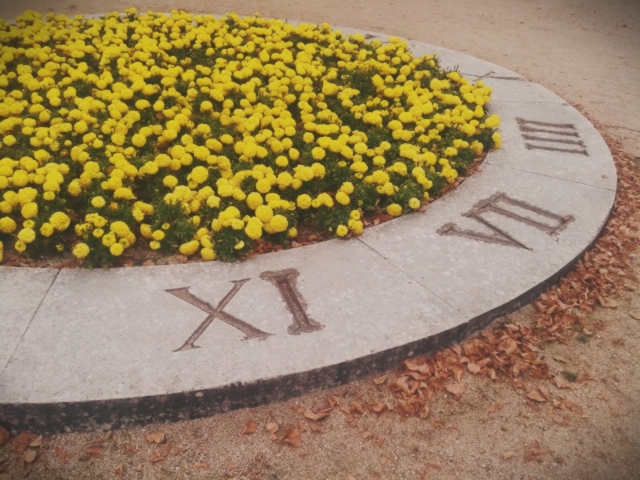The image showcases a circular flower bed, with only the top half visible in the frame. The flower bed appears to be constructed from concrete, divided into equally spaced sections resembling bricks. Each brick features Roman numerals and numbers, notably displaying 'VIII', 'IX', and possibly 'IV' or 'VII'. The central area is vibrant with flowers boasting either green or yellow petals and lush green stems. Surrounding the flower bed, there is a considerable amount of additional concrete pavement, scattered with an abundance of brown leaves that look as though they have been swept up against the structure by the wind.